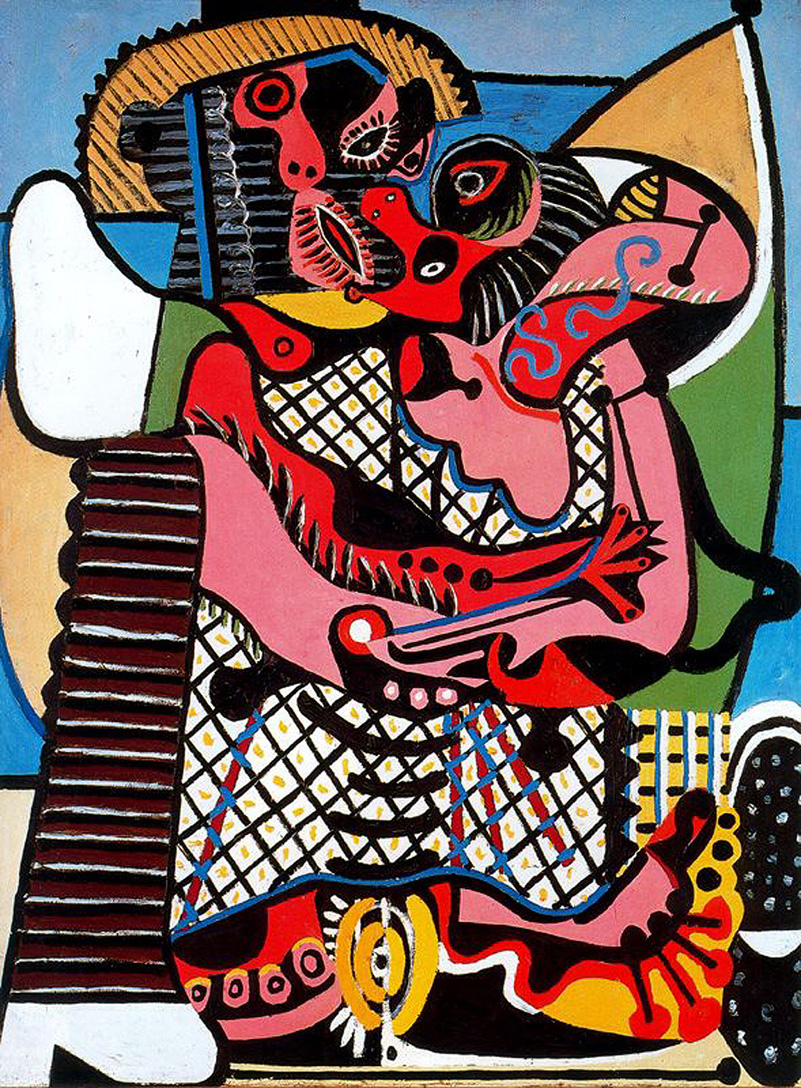The abstract painting is a vibrant and busy piece, bursting with ornate details and vivid colors including blues, reds, yellows, blacks, and whites. The background features light to medium blue hues in the upper right and upper left corners. Central to the image is a highly stylized and contorted figure of a person with a face that appears turned sideways. The face has multiple eyes and a large, arcing nose with a mix of pink, yellow, white, and black colors, and red highlights underneath.

The figure's hair, depicted in gold, appears at the back of the head, and the bottom of the hair blends into blue hues. The head also reveals an inner face-like structure with distinguishable features such as an eye and ear-like shapes. The person is adorned with a quilted pattern in their clothing, featuring black horizontal lines and interspersed with red lines. 

The arms are wavy and patterned, reminiscent of an elephant's trunk, while one leg, curving horizontally to the left, is depicted with a white boot. Another leg appears sideways with black and white stripes, and nearby, two pairs of black shoes with white polka dots are positioned vertically opposite to each other.

Below the waist, the figure's attire continues with a dress-like section marked with red, white, and black horizontal square rectangles and lines. The feet underneath resemble toes, with one foot featuring black pins protruding from it and a small golden circle section nearby. The abstract image culminates with additional black elements at the bottom, possibly stone-like, and a large green section in the background, contrasting with a white area on its left, further enhancing the painting's elaborate and surreal nature.